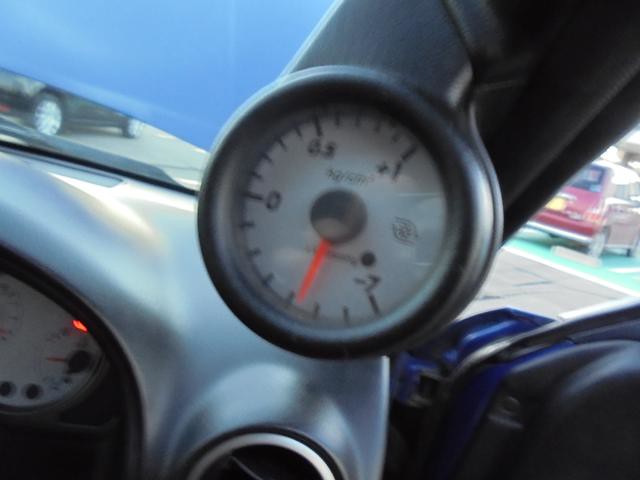The image depicts an OEM (Original Equipment Manufacturer) analog gauge, likely a vacuum or boost pressure gauge, located within a car's dashboard. The gauge features a white face with a red needle, scaling from +1 at the top to -7 at the bottom. Currently, the needle is pointing to approximately -3. Despite the image being slightly blurry, it is clear the gauge is an integral part of the car's instrumentation, implying it is not an aftermarket addition. The dashboard is visible behind the gauge, showing a red warning light illuminated and air vents for climate control. Additionally, the car's hood appears to be open, as indicated by the lines and light angles.